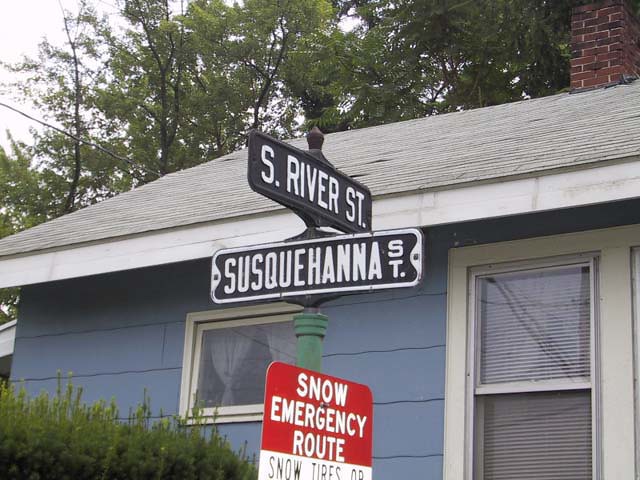A quaint, petite house with a shingled roof and a brick chimney positioned in the top right corner of the photo. The light blue exterior of the house is set against a backdrop of tall, lush trees that span the entire width of the image, starting near the chimney and extending to the left edge. The front yard is adorned with overgrown bushes in need of trimming. A square window with two white curtains, elegantly tied in the middle, adds charm to the house. The front door is framed with white trim, and a red sign marked "Snow Emergency Route" with white letters stands in front of it. Nearby, there are two street signs: one reading "Susquehanna Street," with white letters on a black background and a white outline, and another reading "South River Street," with white letters on a black background but without an outline.